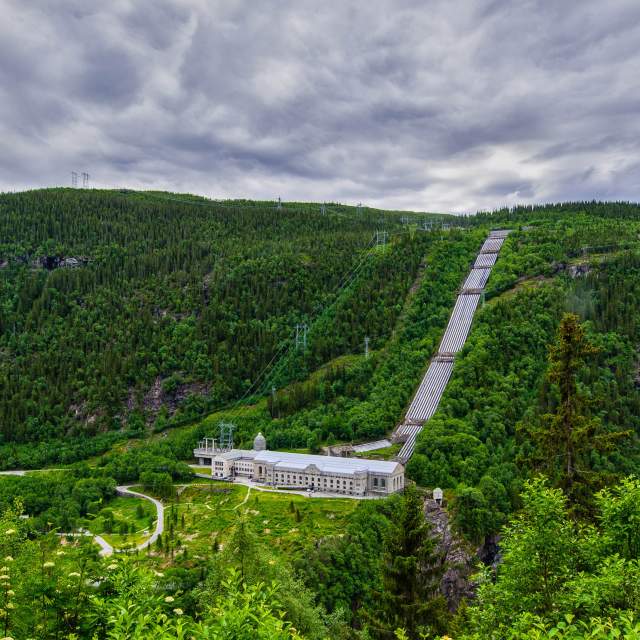The photograph captures a vast, lush green hillside dotted with numerous evergreen trees, painting a scene rich in varying shades of green from a higher vantage point. Dominating the landscape is a long, white building with numerous dark, empty-looking windows, suggesting either an abandoned or seldom-used industrial function. This building sits majestically towards the base of the hill, reminiscent of modern or industrial architecture, and is complemented by a flat roof and a tall, rounded tower at its rear.

Surrounding the building, a network of paved roads meanders through the forested area, enhancing the sense of infrastructure amidst the natural setting. Additionally, high-voltage power lines extend down the mountainside, indicating the presence of significant electrical activity which seems to be emanating from the building. This is coupled with an array of what appears to be solar panels or striped piping structures climbing the hill directly among the trees, further hinting at a possibly functional facility, such as a power plant. Above, the sky is cloud-filled, casting a whitish-blue hue across the scene, enhancing the dramatic and somewhat surreal atmosphere of the photograph.